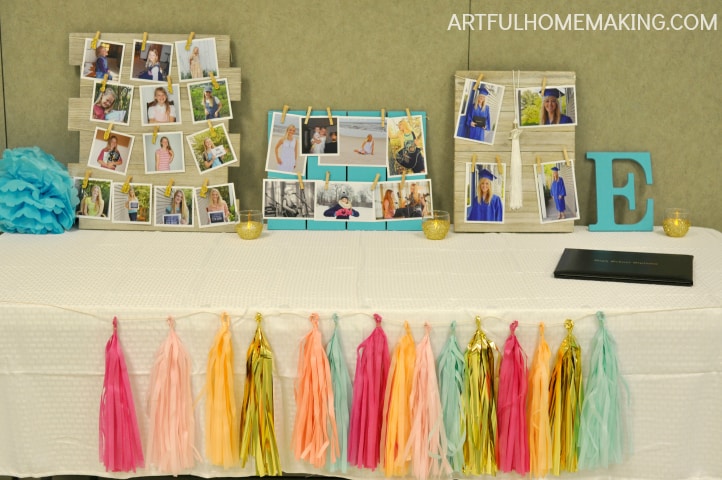This image appears to represent a decorative setup likely featured on a website, as indicated by the off-white text "artfulhomemaking.com" in the upper right corner. The scene features a long banquet table draped in an off-white tablecloth, set against a sponge-painted gold wall. Adorning the front of the table are colorful tassels in shades such as pink, light pink, peach, shiny gold, baby blue, and hot pink, arranged in a decorative fashion.

On the tabletop, three personalized boards serve as collages. The first board, wooden and possibly light blue, displays 13 photographs clipped on with paperclips. The second board, a beige wooden surface, features four graduation photos. The third board, also wooden and blue, holds several more photographs. To the right of these boards sits a blue wooden letter "E" and three lit votive candles that have a golden hue. Additionally, a black closed notebook is placed on the table.

Also noticeable on the table is a collection of decorative string tassels in various colors like pink, peach, yellow, green, blue, and turquoise, which seem to be used almost like pom-poms or party favors, adding a festive touch to the overall arrangement.